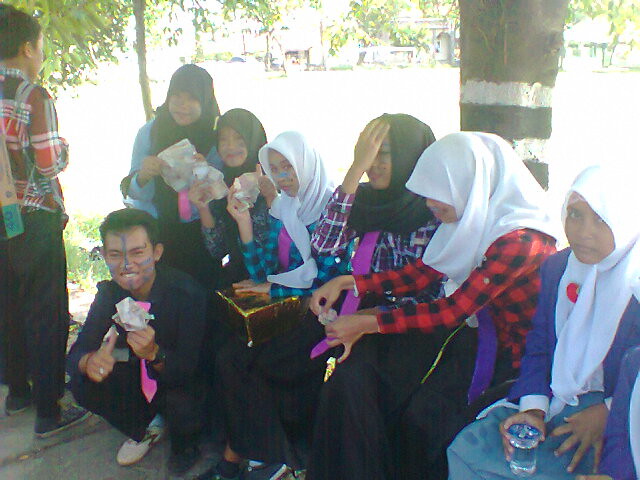In the image, a group of girls, most likely school-aged or young adults of Southeast Asian descent, are sitting under an outdoor overhang. They are all dressed modestly, with several of them wearing black or white headscarves (hijabs) and long black dress-like pants. Some of the girls display blue face paint and wear sashes. They appear to be participating in an event involving eating and drinking, as one girl is holding a glass of water, and another has a yellow box on her lap.

Two boys are present in the image. One is kneeling beside the girls, looking at the camera and cheerfully giving a thumbs up. He wears a black business casual outfit with a pink tie and also has face paint. The second boy is partially visible on the left side of the group, standing and facing away, with only his profile captured in the frame. 

The setting appears to be a sunny park, with tall trees and green leaves visible in the background. The sunlight is bright, creating a somewhat blown-out effect in parts of the image. The girls seem a bit embarrassed or hesitant, adding a candid feel to the photo.